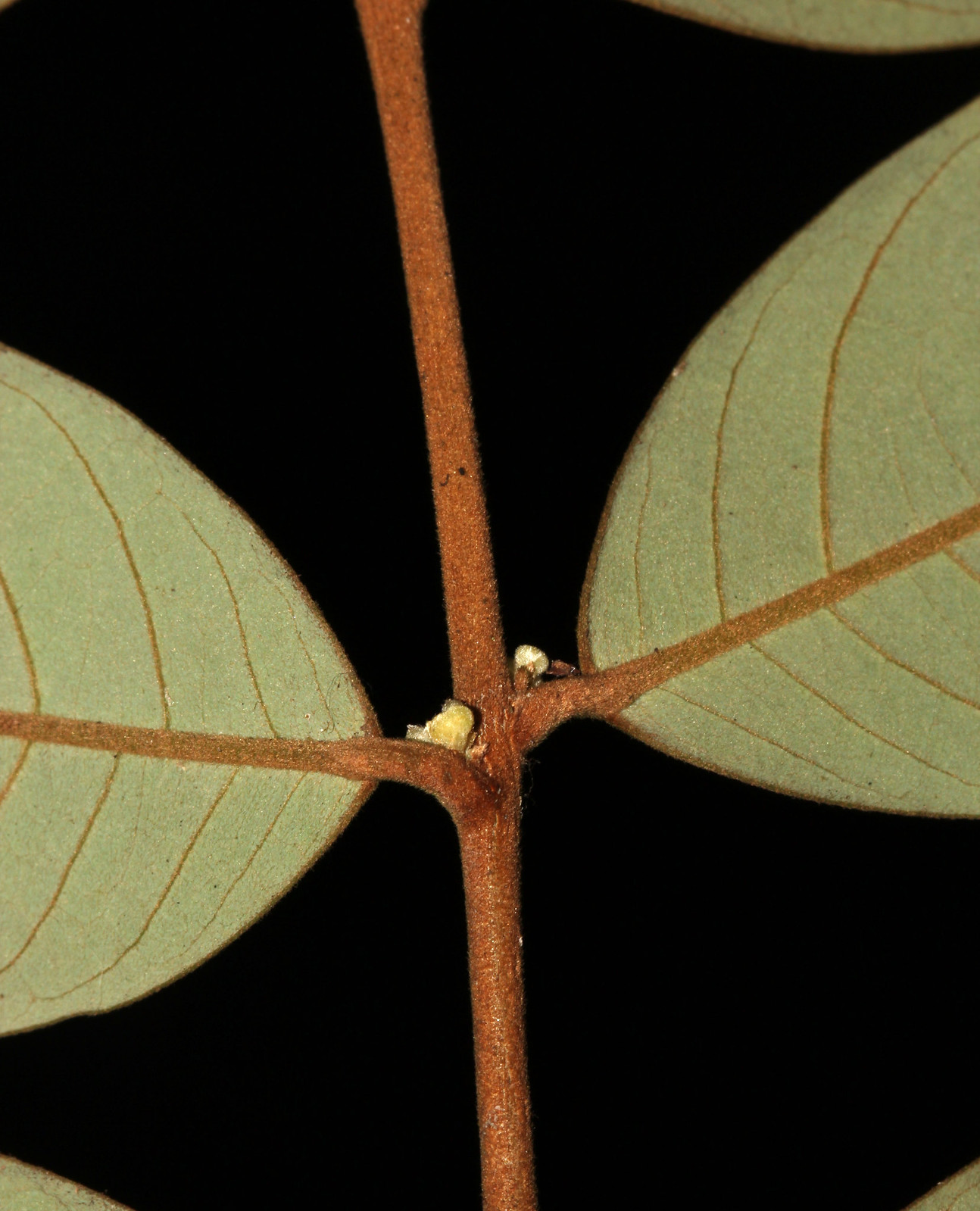This extreme close-up photograph showcases the underside of a plant stem against a pure black background, devoid of any extraneous details. The central brown stem extends vertically from the top to the bottom of the image, splitting into two smaller branches that diverge to the left and right. The light green leaves, primarily showing their undersides, emerge from these branches and dominate the left and right edges of the frame. The leaves feature small chocolate brown veins, and the extreme zoom reveals a slight fuzz on both the stem and leaves. At the center of the stem's split, slightly below the middle of the image, there is a yellow object, which might be a bud, a bit of fungus, or an extremely small animal, but its exact nature is indeterminate at this resolution. Additionally, a couple of black dots appear on the stem just above the center, likely a result of the extreme close-up perspective.